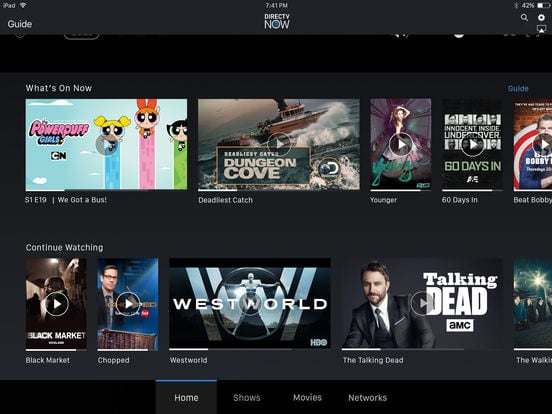The image displays a user interface screen from DirecTV Now with a predominantly black background. At the top center of the screen, small white text shows the time "1:41 p.m." and the DirecTV Now logo. To the left, there's the word "Guide."

Underneath this heading, the section labeled "What's On Now" features thumbnails of current shows. The first thumbnail has a blue background with three cartoon characters with large black eyes and tiny white dots. This thumbnail is labeled "Powerpuff Girls" in pink text, with the channel "CN" (Cartoon Network) beneath it.

Next to this, there is an image labeled "Dungeon Cove," featuring a ship on the ocean. Beside it is another thumbnail for the show "60 Days In," with the network "A&E" noted below it. Next to this, there is a clickable white option labeled "Continue Watching."

The "Continue Watching" section includes several options. The show "Black Market" is listed, followed by "Chopped," and then "Westworld." The "Westworld" thumbnail is the largest, featuring a prominent blue 'W' on it. Adjacent to it is a thumbnail for "The Talking Dead," showing a man in a suit with a serious expression. Under "The Talking Dead," there's a white box with the letters "AMC," indicating the network.